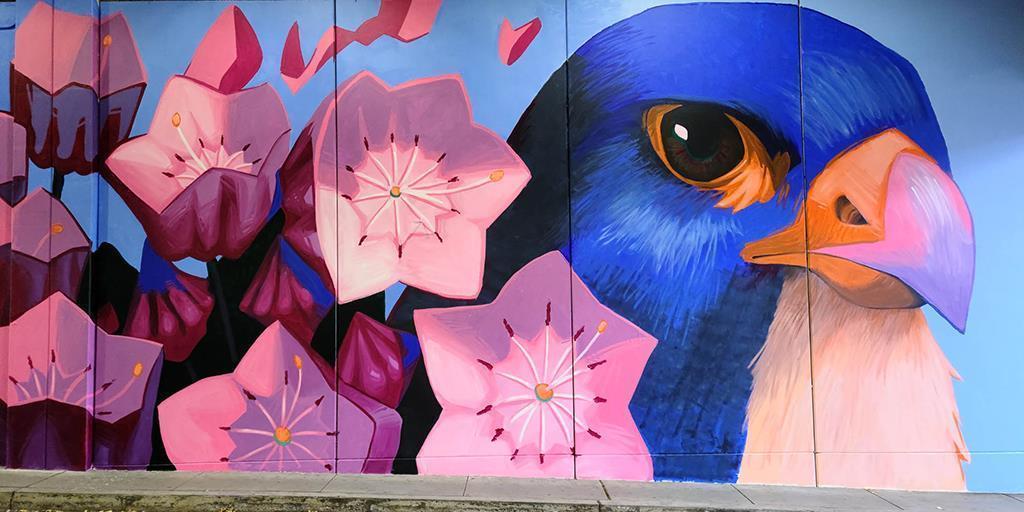This detailed rectangular drawing on five panels primarily depicts a large bird's face and vibrant flowers, with the left side slightly cut off. The bottom three and a portion of the fourth panel feature clusters of flowers; their petals are dark pink at the base and transition to light pink toward the centers, surrounded by white stamens. Notably, some stamens have yellow or red tips. Above the flowers is a clear blue sky, occupying the same panel space.

On the right-hand side, a striking bird's head takes up the remaining two and a half panels. This avian subject boasts a vivid blue head and a large, dark brown eye, highlighted by a black pupil and encircled by a light orange hue. The bird's substantial, curved beak is white, with an orange area wrapping under and around it, including the nostril. The visible chest of the bird is white, which becomes obscured by what appears to be a gray line – possibly the image frame – although the exact boundaries remain unclear due to the partial cut-off.